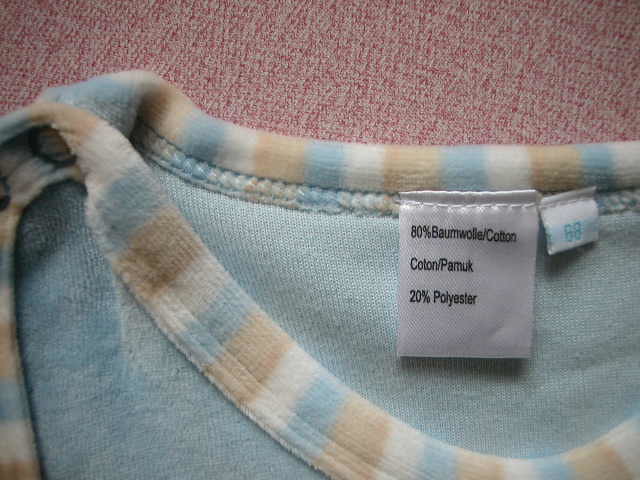This image depicts a close-up view of a soft shirt, likely a piece of velour clothing, laid out on a fabric-covered surface. The shirt predominantly features a light blue color with subtle white, beige, and very light brown stripes adorning its collar. The fabric background appears to be a blanket in shades of pink and cream. The collar also showcases this mix of colors, providing a soft and visually soothing contrast. The shirt includes a label indicating its composition: 80% cotton (referred to as 'Balmwool' and 'Pamuk' in different languages) and 20% polyester. Additionally, the image shows a size tag marked as '68'. The close-up nature of the photograph is detailed enough to see the stitching of the fabric, though it remains slightly blurry. Overall, the cozy and comfortable qualities of the shirt stand out against the patterned and colorful background.